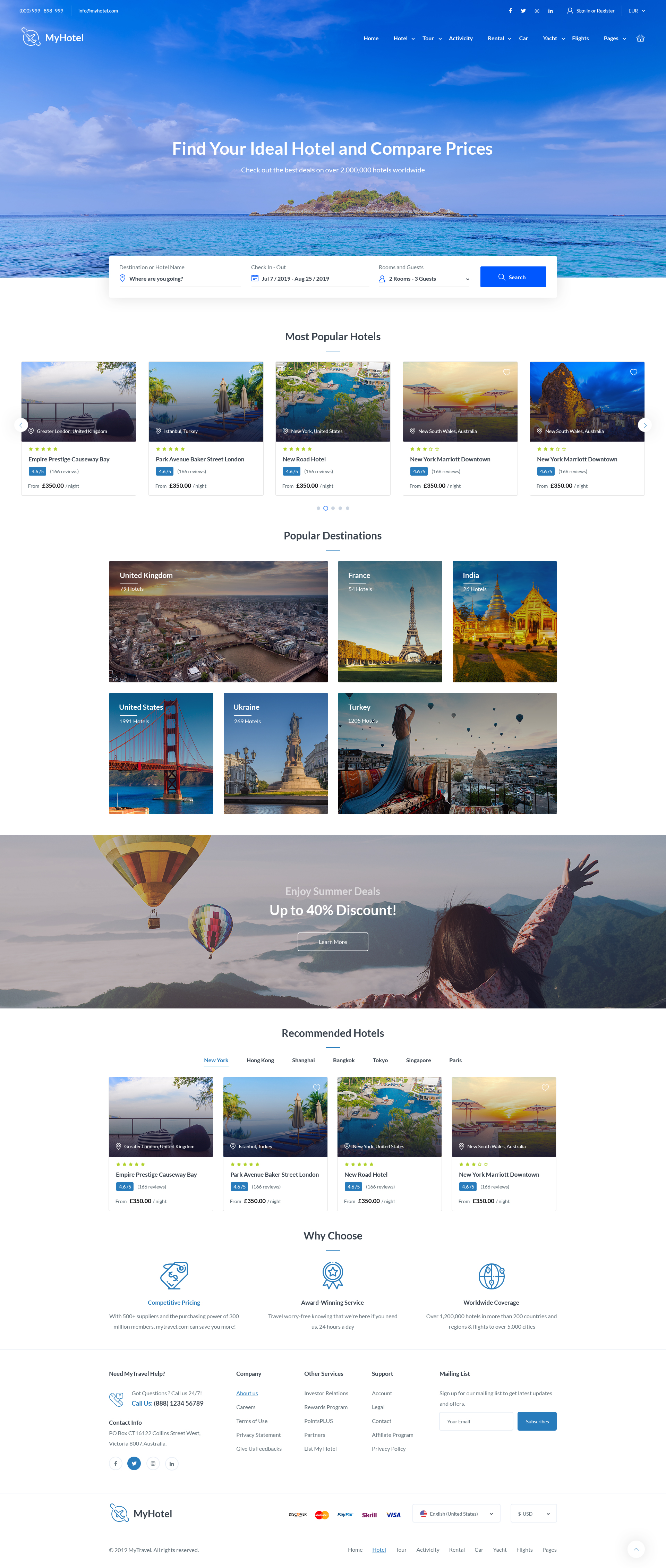This is a detailed screenshot of the "My Hotel" website. The screenshot is small and requires zooming in for clarity. At the top left corner of the website, you can observe the logo and icon, which features an airplane flying diagonally upwards to the left with a planet encircling it, creating a rather unusual visual. Next to the logo, the contact details are prominently displayed, including a phone number, "XX999898999," and the email address, "info@myhotel.com."

On the top right corner, several navigation tabs are listed: Home, Hotel, Tour, Activity (which is misspelled as "Acticity"), Rental, Car, Yacht, Flights, and Pages. There's also an additional logo resembling a face, potentially indicating a chatbot feature. Additionally, various social media icons for Facebook, Twitter, and Instagram can be found in the top right section, providing quick links to their respective platforms.

The center of the page is dedicated to guiding users in finding and comparing prices for their ideal hotels, emphasizing the website's core service.